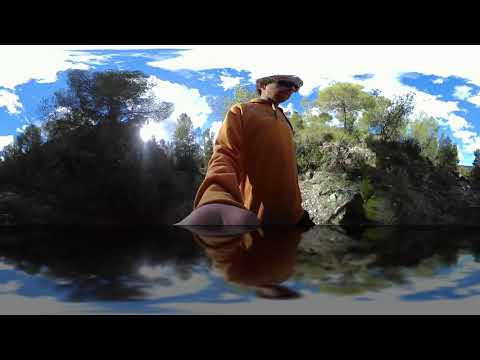In this highly detailed panoramic photograph, a young man takes a selfie using a reflective device, likely a smartphone or tablet, held in his right hand. He is dressed in a long-sleeved pullover hoodie with black and yellow drawstrings, which is orange in color. The hoodie has its hood down, revealing his blond hair and sunglasses, adding a casual yet trendy element to his look. The man is visible from the waist up, seemingly standing in the wilderness surrounded by thin trees clothed in green leaves and a landscape peppered with various gray rocks and boulders.

The background presents a beautiful natural scene under a light blue sky dotted with thick white clouds. The lighting suggests daylight, with the sun casting noticeable shadows on the ground and rocks, indicating the sun is either low in the sky during late evening. The trees on the right side of the image reflect sunlight, while those on the left are in shadow, creating a contrasting, serene ambiance. The panoramic nature of the image introduces a slight distortion, giving an interesting depth to the entire composition, enriching the visual narrative with its unique perspective.